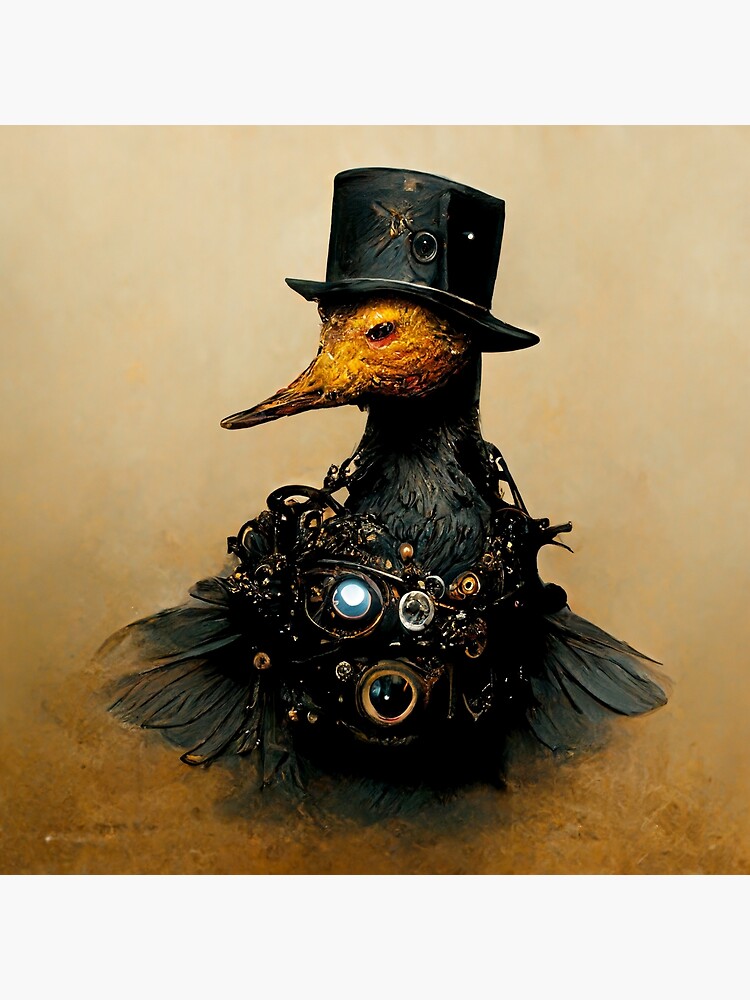The image depicts a steampunk-inspired, fantastical bird creature with an elaborate appearance. The bird, possibly carved from wood, is adorned with detailed metalwork and jewels that complement its intricate design. Its body is predominantly black with elements of rusty metal, grayish-green feathers, and a grayish-green body. The face of the bird is a distinct golden yellow, accentuated by a gold mask covering its eyes, giving an impression of bleeding dark irises.

Perched atop its head is a striking top hat resembling a pork pie hat, accessorized with three prominent jewels and traditional steampunk gold decorations, including a noticeable white dot near the back. This hat also features additional baubles and feathers reminiscent of a peacock's tail.

The bird stands against a distressed, muted yellow-brown background designed to evoke an antique or dusted appearance. Various jewels and wires adorn the creature's body, from an opal-like stone on the left breast to a trail of dark, shiny jewels, all connected with intricate cabochon style jewelry, creating a cohesive and visually captivating steampunk aesthetic. The overall ambiance of the image is a blend of oddity and charm, giving it a unique yet endearing appeal.